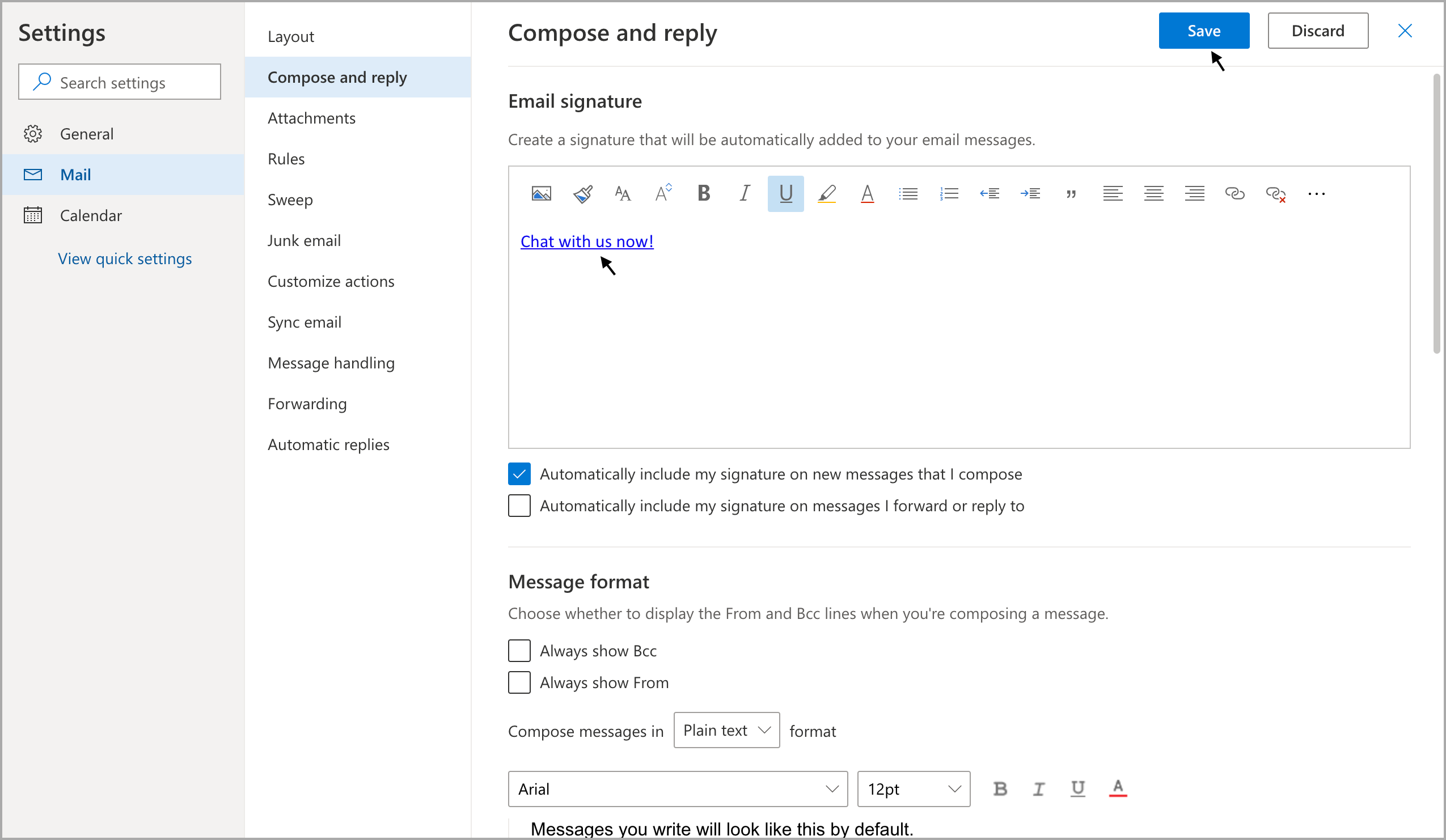The image captures a screenshot from a website featuring an email settings interface. The background is primarily white, with the left side dominated by a gray rectangular panel containing various configuration options. These options include General, Mail, Calendar, and Quick View settings. Adjacent to this panel is a broader section detailing specific settings categories such as Layout, Compare and Reply, Compose and Reply, Attachments, Rules, Sweep, Junk Email, Customize Actions, Sync Email, Message Handling, Forwarding, and Automatic Replies.

In the main content area, the "Compose and Reply" setting is selected, indicated by the highlighted category at the top. The central portion of the screen is focused on the "Email signature" feature. A description beneath this heading explains, "Create a signature that will be automatically added to your email messages." 

There is an interactive element labeled "Chat with us now," providing users with a clickable link for live support. A black arrow is pointing towards the section that allows users to set up their email signature. Specifically, there's a checkbox labeled "Automatically include my signature on new messages that I compose," which is ticked. 

No other checkboxes are selected, yet another black arrow directs attention to the "Save" button, highlighted in blue at the top of the interface.